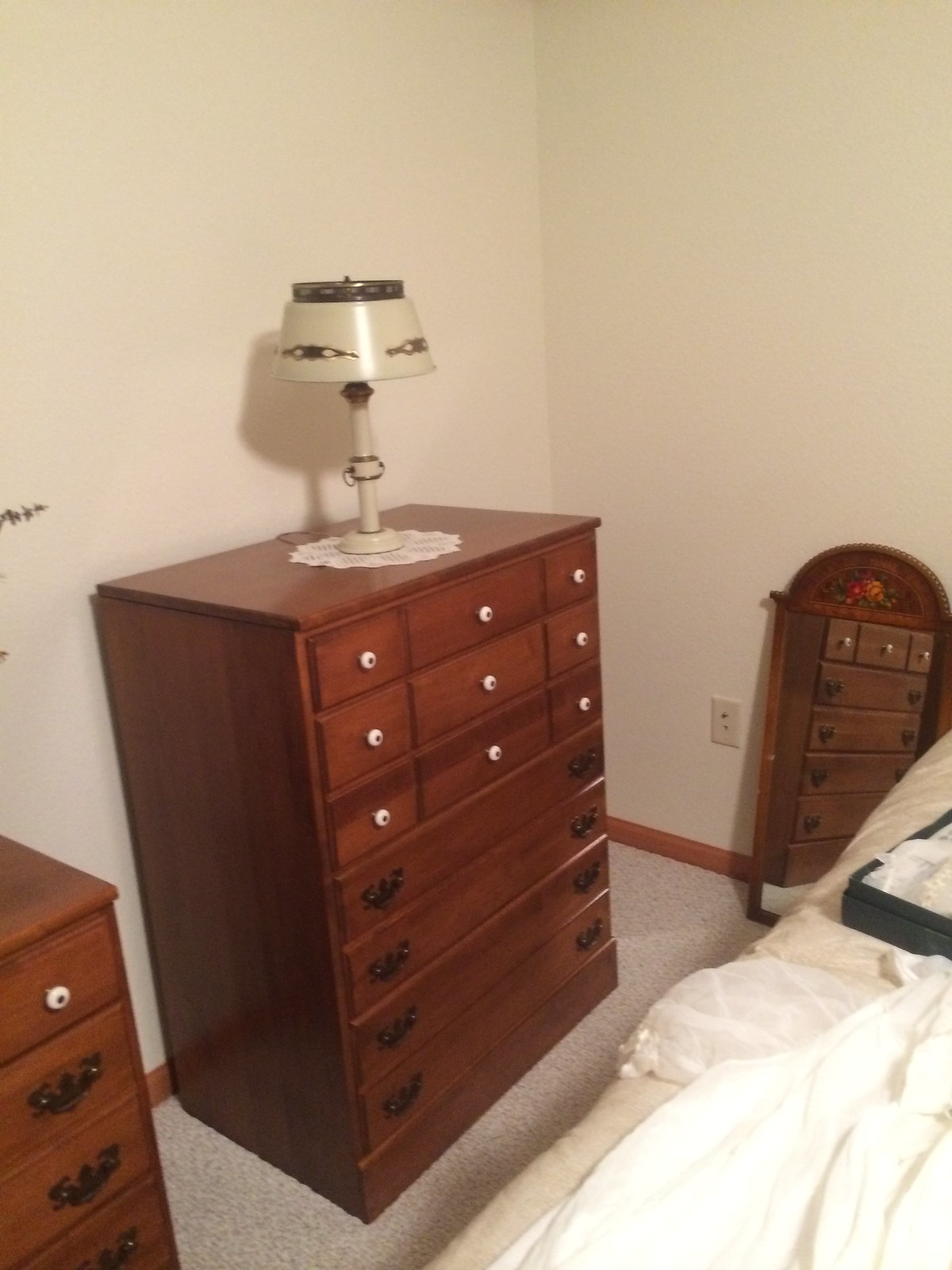This detailed bedroom photo showcases a large dark brown dresser with a reddish tint, featuring seven rows of drawers. The top three rows each have three columns of drawers equipped with white knobs, perfect for organizing smaller items such as jewelry. The bottom four rows sport black metal handles on either side of each drawer. On top of this dresser sits a white doily and a cream-colored lamp with a subtle design.

Adjacent to this dresser is a slightly smaller, equally dark brown cabinet with a similar varnish. It features a mix of drawer types, including one with a round opener on the top right. In the corner where two white walls meet, the room's beige rug flooring is visible along with a tan floor runner.

To the right of the dresser is a white bed with a cream-colored bedspread, on which rests a blue suitcase partially packed with a white item. A mirror, with a brown wooden frame, reflects the dresser adding depth to the room. The setup hints at practical organization and comfort, highlighted by small details such as an Ethernet port and the subtle decor of the cream-colored lamp.